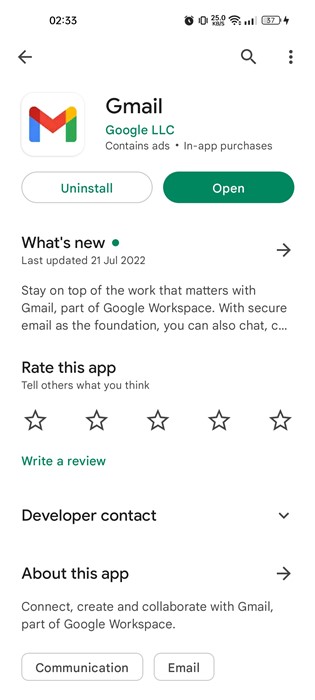The image displays a mobile phone screen with a white background. The time is shown as 2:33, along with an alarm clock icon. The battery indicator shows either 37% or 57%, but most likely 37%, and includes a charging symbol (a thunderbolt icon). At the top left, there's a left arrow and a magnifying glass icon, followed by three vertical dots representing additional options.

The screen displays the Gmail app page on Google Play Store. The app is developed by Google LLC, noted in green text, and it contains ads and in-app purchases. Below the app's name, two oval buttons are present: one white with green text "Uninstall" and a green one with white text "Open".

A section titled "What's new" with an accompanying green dot and right arrow indicates updates. The last update date is listed as 21 July 2022. The description reads: "Stay on top of the work that matters with Gmail. Part of Google Workspace with a secure email as the foundation. You can also chat and have (...)".

There is an invitation to rate the app with five stars and a prompt in green text to "Write a review." Below, there are options for "Developer contact" with a down arrow and "About this app" with a right arrow. The description below emphasizes connecting, creating, and collaborating with Gmail as part of Google Workspace. Finally, two rectangular buttons categorize the app under "Communication" and "Email."